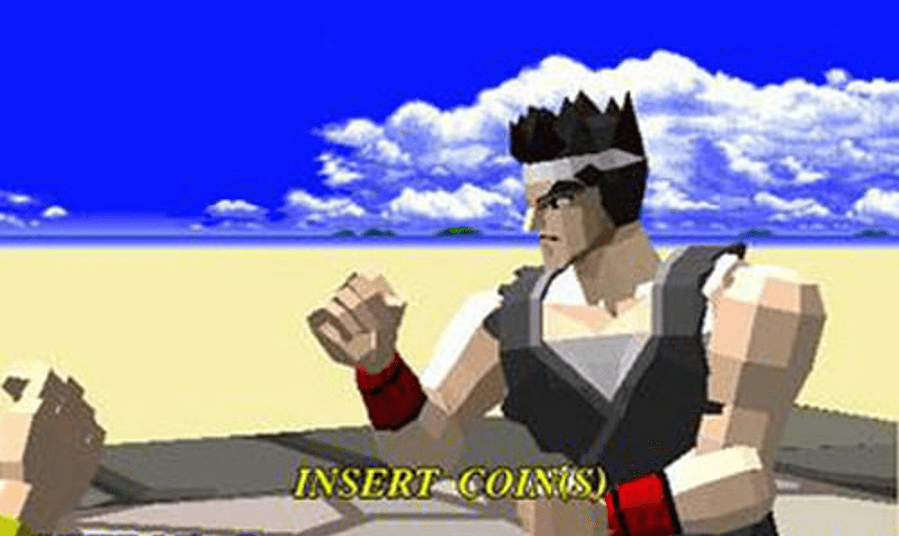This image is a screen from a vintage arcade video game, featuring a pixelated, 8-bit character reminiscent of old-school fighter games. The character stands centrally to the right, immersed in a scene with a vivid blue sky dotted with fluffy white clouds, a deep blue waterline, and a sandy-beige horizon. The figure itself is composed entirely of rigid angles, exuding a boxy and primitive computer graphic style.

Adorned with a spiky black mohawk and a white headband, the character sports thick, bushy eyebrows, a prominent beaky nose, and muscular arms accentuated by red wristbands on both wrists. He wears a dark gray and black vest while adopting a fierce expression, his gaze directed off to the side. His stance is dynamic, with one fist raised and the other lowered. In front of him, a gray, square-patterned table is visible.

Overlaying the lower part of the screen, bright yellow text reads, "Insert Coins," highlighting the gaming context. Overall, the image captures the essence of a nostalgic, 8-bit arcade fighting game.